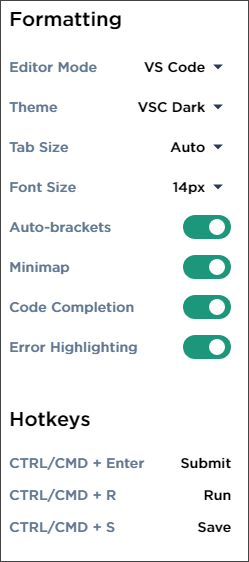**Image Caption: Detailed Description of a Formatting Settings Menu**

The image displays a rectangular area with a white background, framed by a very thin black border. Positioned towards the upper left of the image, bold black uppercase letters spell out "FORMATTING". The image appears slightly distorted, adding an element of visual skew.

Below this header, the settings menu is divided into several sections, each delineated with gray bold subtitles and corresponding black bold settings to the right. The descriptions are as follows:

1. **Editor Mode:** 
   - Subtitle: "Editor Mode" in gray bold lettering.
   - Setting: "VS CODE" in black bold uppercase letters, followed by a drop-down menu indicated by an arrowhead pointing downwards.

2. **Theme:**
   - Subtitle: "Theme" in gray bold lettering.
   - Setting: "VSC DARK" in black bold uppercase letters, with a corresponding drop-down menu to its right.

3. **Tab Size:**
   - Subtitle: "Tab Size" in gray bold lettering.
   - Setting: "AUTO" in black bold lettering, accompanied by a drop-down menu option.

4. **Font Size:**
   - Subtitle: "Font Size" in gray bold lettering.
   - Setting: "14px" in black bold lettering, with a drop-down menu symbol to the right.

5. **Auto-Brackets:**
   - Subtitle: "Auto-Brackets" in gray bold lettering, without any space between the words.
   - Setting: A toggle option indicated as turned on.

6. **Mini-Map:**
   - Subtitle: "Mini-Map" in gray bold lettering.
   - Setting: A toggle option, which is activated (on).

7. **Code Completion:**
   - Subtitle: "Code Completion" in gray bold lettering.
   - Setting: An active toggle option.

8. **Error Highlighting:**
   - Subtitle: "Error Highlighting" in gray bold lettering.
   - Setting: A toggle option turned on.

Each setting is neatly aligned, with the subtitles on the left and corresponding settings on the right, providing a comprehensive overview of various formatting options available in the editor.